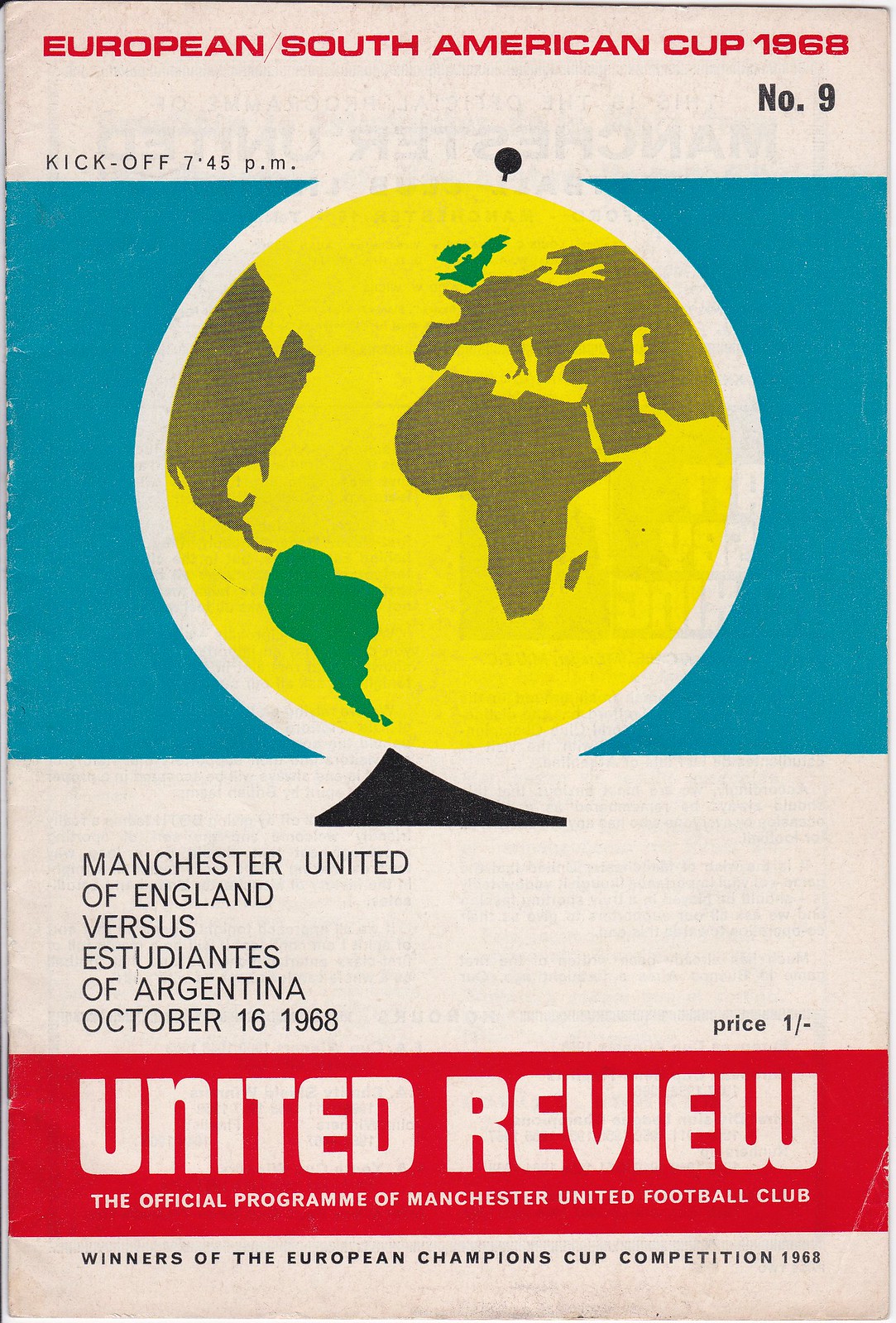The cover design of this sports program, predominantly white, showcases the event "European/South American Cup 1968" in red text at the very top. Just below this title, "NO9" is printed in black. A prominent blue banner runs below, featuring a yellow and green globe depicting highlighted regions of South America and Europe, within a white circle. Directly beneath the globe, a white banner states "Manchester United of England vs Estudiantes of Argentina, October 16th, 1968." At the bottom, a red banner with white text reads, "United Review, the official program of Manchester United Football Club," followed by another white banner declaring Manchester United as the "Winners of the European Champions Cup Competition 1968." The program also mentions the kickoff time as 7.45 p.m. in small text, adding to the detailed layout of the event.